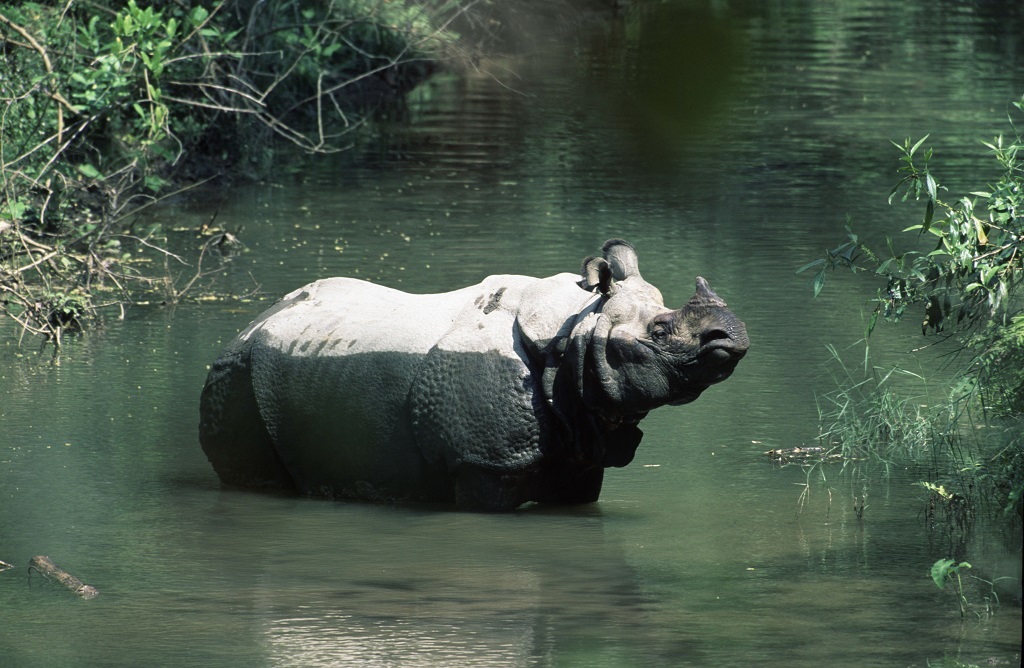This outdoor photo, taken during the day, features a large adult rhinoceros standing in the middle of a calm, green-colored body of water that resembles a lake or stream. The rhinoceros, primarily dark gray and black with a single small horn in front of its nose, is facing right, presenting a profile view. Its eyes are closed and it is illuminated by sunlight that highlights the top third of its body, from the ears to the back, creating a light gray, almost white sheen on its normally scaly skin. The water around the rhino shows slight ripples and a faint reflection of the animal. Surrounding the water, there is vegetation with branches and leaves on both the left and right sides of the image. The foliage on the right appears lush and green, whereas the plants on the left are more sparse, revealing some brownish branches. The rhinoceros' legs are submerged up to their tops, and the composition is balanced by the green shrubs extending from both the upper left and right corners toward the center, framing the majestic creature in its natural habitat.